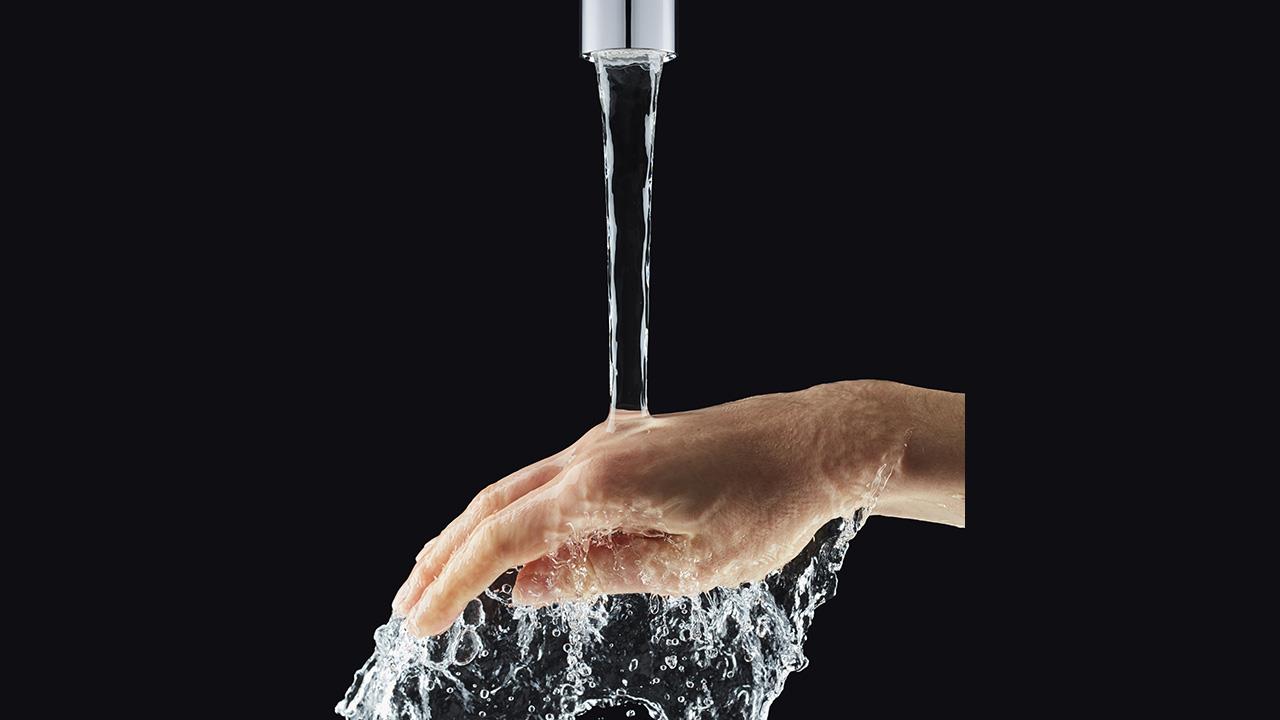In this meticulously staged, full-color photograph with a landscape orientation, a human right hand, Caucasian, is prominently featured being bathed in a clear stream of water from a silver faucet positioned at the top center. The background is entirely black, enhancing the contrast and focus on the hand and water. The faucet's spout, sleek and chrome, is the focal point from which the clear, non-aerated water flows. The water lands precisely on the knuckles of the hand, which is positioned with fingers pointing left and slightly downward, the thumb extending forward and wrist subtly bent. The hand, emerging from the right side into the center of the image, wears a black shirt that melds seamlessly into the black background. Below the hand, the water splashes and disperses in different directions, creating dynamic reflections and a cascade that adds to the realism and depth of the photograph.